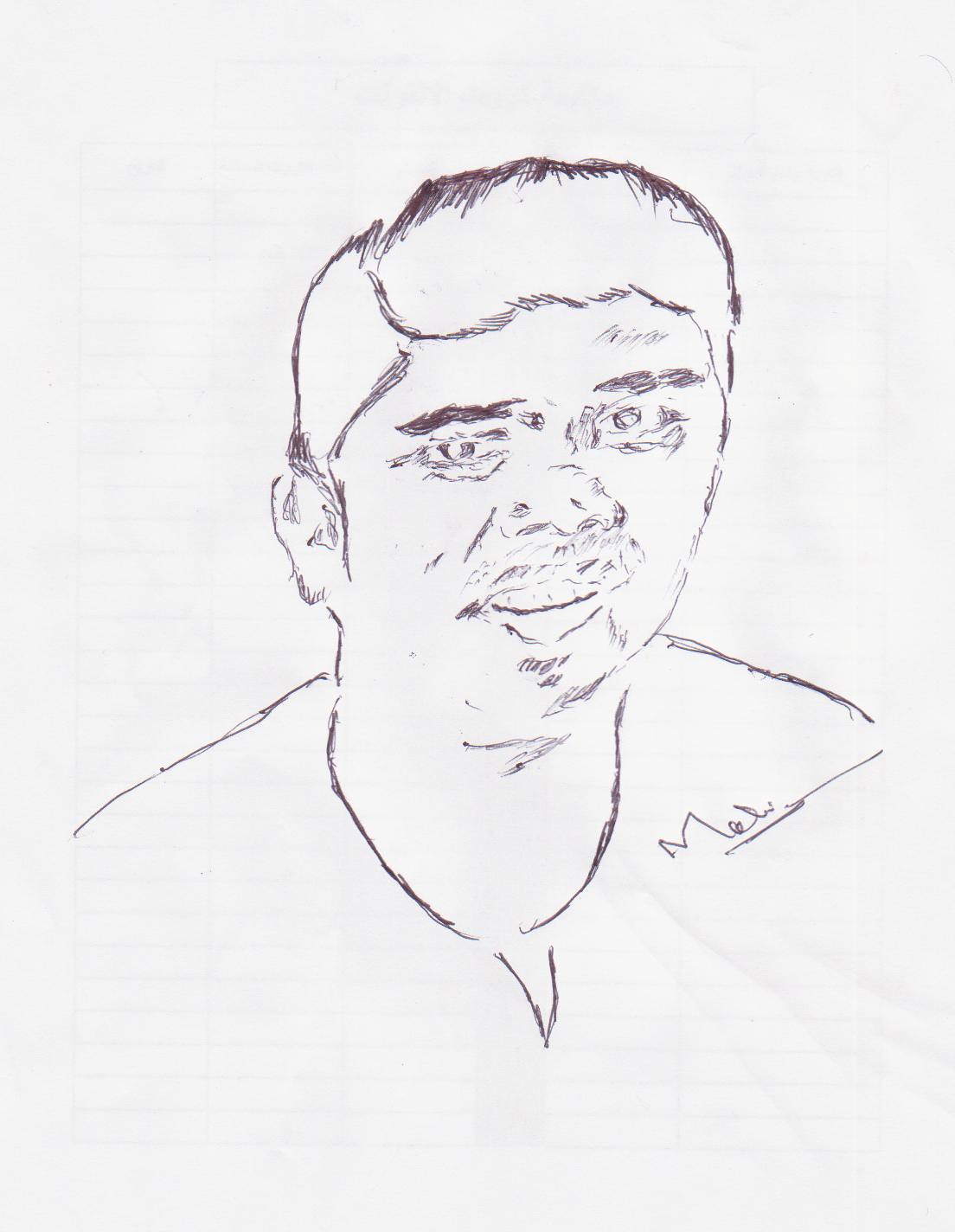A black-and-white sketch depicts a person, likely a man, characterized by the presence of facial hair. This minimalist illustration focuses on the face and upper body of the subject, with facial features drawn in an open, doodle-like style that leaves room for interpretation. The man's mouth is open, revealing his front teeth, possibly suggesting a smile. Other discernible features include a visible nose and faint bags under the eyes. The drawing is signed by the artist with a partially legible signature, which appears to start with the letters "MOA," and is underlined for emphasis.